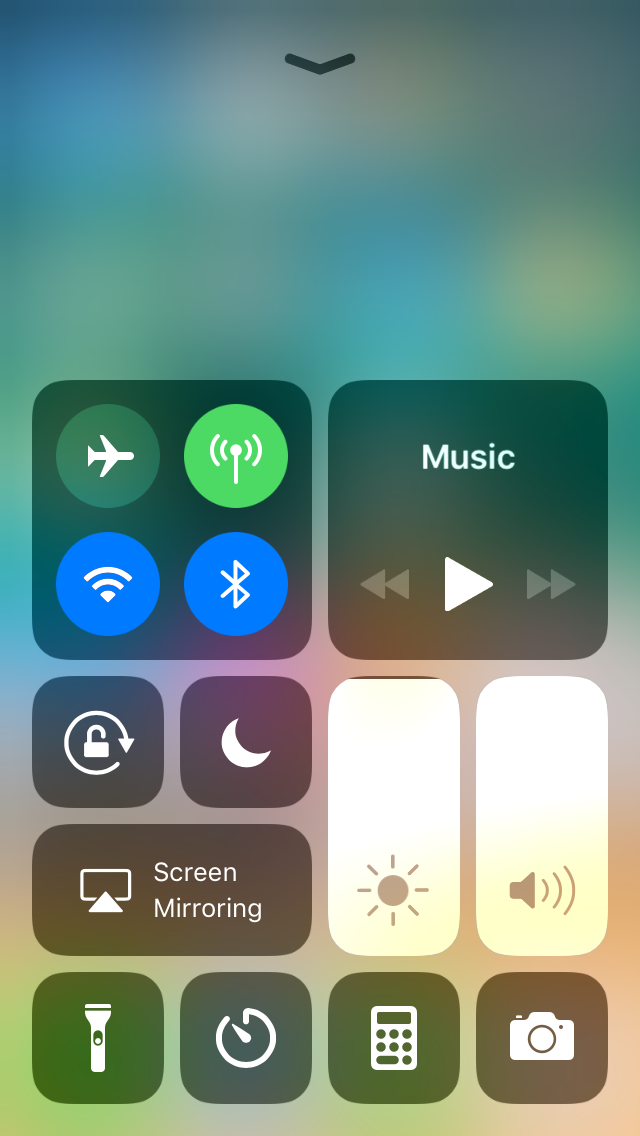This screen capture from an iPhone in portrait mode, showing a detailed view of the Control Center, fills the lower two-thirds of the screen. The capture highlights several key control settings. At the top of the screen, a black arrow points downward, indicating the option to drag the menu bar back to its hidden position.

In the upper left quadrant, a square housing four icons shows that Wi-Fi, Bluetooth, and the green cellular connectivity toggle are turned on, while Airplane Mode remains inactive. To the right of this, another prominent square contains the Music control panel, featuring a white play button flanked by skip backward and forward buttons.

Below the Music panel, two vertical sliders for brightness and sound are displayed, both set to their maximum levels. Directly to the left of these sliders are three small icons for lock screen, night mode, and screen mirroring, none of which are activated.

At the bottom of the screen, four essential controls are visible from left to right: flashlight, clock, calculator, and camera. The top of the screen is occupied by a blurred-out image of the phone's background, providing a subtle aesthetic touch to the interactive elements below.